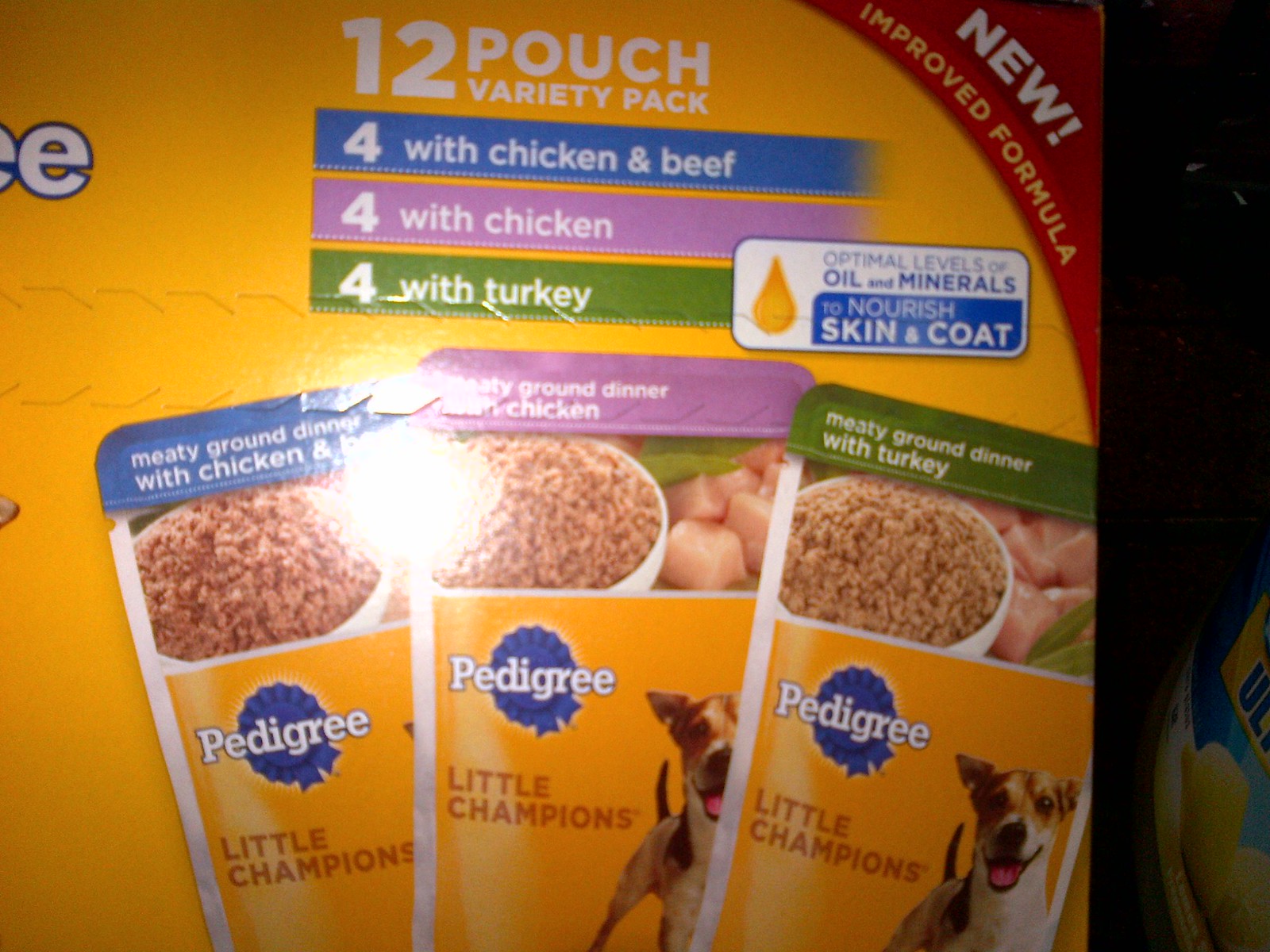The image features a close-up photograph, captured with flash, of a yellow Pedigree dog food box, slightly out of focus due to the camera's proximity. The box, prominently placed in the center and slightly to the left, is illuminated with a bright flash reflecting off its surface, creating a ball of light in the middle and shadows to the far right. The box is identified as a 12-pouch variety pack with white block letters indicating "Pedigree" accompanied by a blue ribbon. The top right corner of the box has a red triangle with text in white that reads "NEW! Improved Formula." Below, the white text states "12 Pouch Variety Pack."

The box showcases three flavor varieties, delineated by different colored stripes: blue for "Four with Chicken and Beef," lavender for "Four with Chicken," and avocado green for "Four with Turkey." Below these stripes, there are three small photographs of the dog food pouches, each depicting the wet dog food in a bowl. Beneath these images, the text "Little Champions" appears in dark orange on a plain orange background, next to a smiling small dog that resembles a Jack Russell Terrier with brown ears and a pink tongue hanging out. The Pedigree logo—a blue ribbon with "Pedigree" written in white block letters—is also visible beside the dog. Additionally, you can spot squiggly lines on the box, indicating an easier open section.